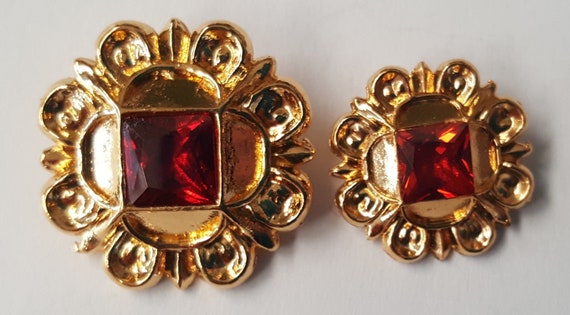This photograph showcases two exquisite pieces of gold jewelry, likely brooches, set against a light gray background. Both pieces are identical in design but differ in size, with the one on the left being larger and the one on the right about half its size. Central to each brooch is a prominent square-shaped gem, likely a red ruby, which is encircled by symmetrical gold half-circles that give the impression of flower petals. The ornate design extends outward in a pattern of eight semi-circles interspersed with lines, creating a radiant, sun-like appearance. The larger brooch casts a light shadow to its right, with the smaller brooch angled slightly toward the right, enhancing the visual interest. The intricate craftsmanship and repeated floral motif highlight the elegance and harmony of these identical yet variably sized pieces.